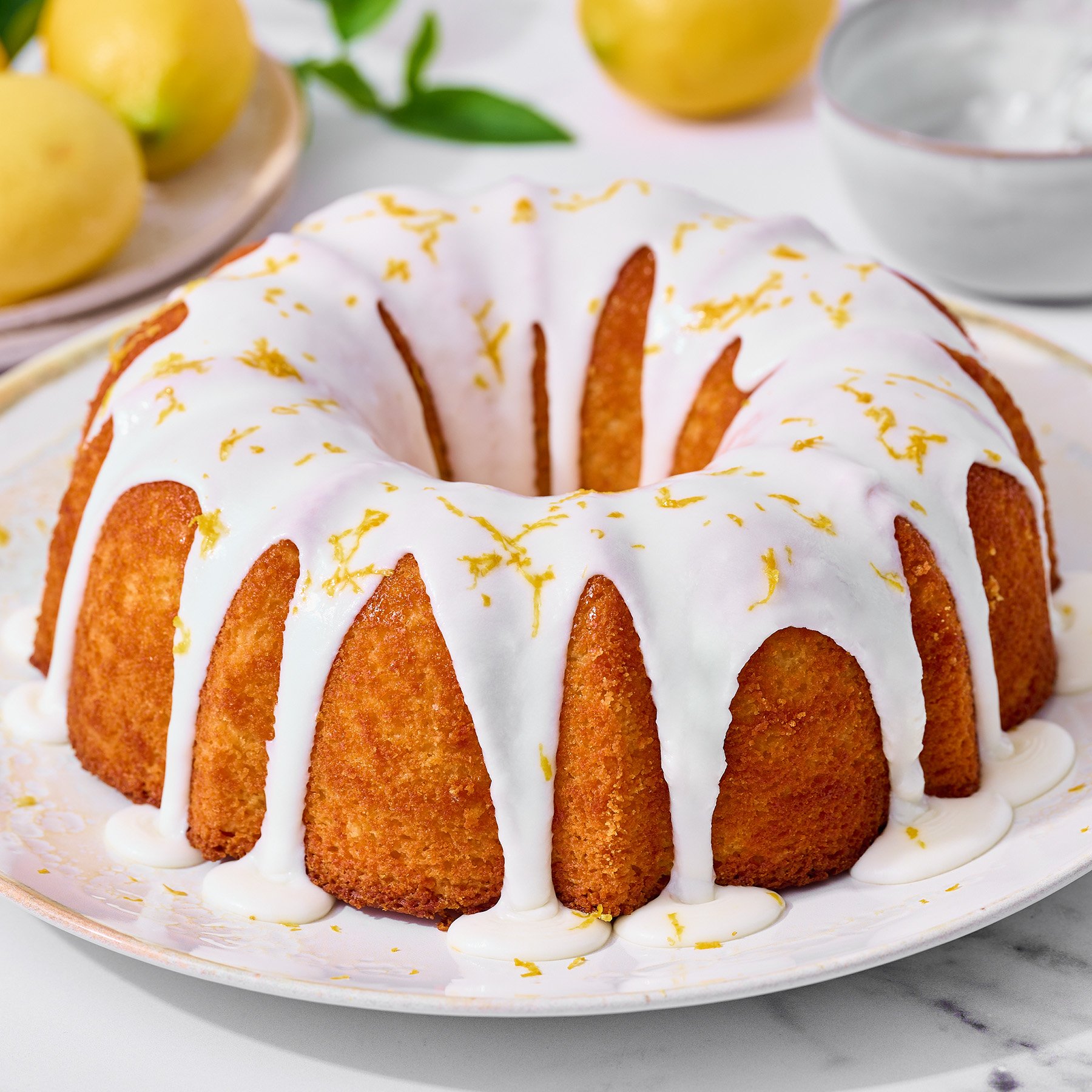The photograph captures a professionally styled image of a lemon Bundt cake, positioned prominently in the center of the frame. The cake, a light orange-brown hue, is adorned with a glossy white icing that cascades elegantly over its sides, forming small pools and drips that reveal portions of the sponge beneath. A generous sprinkling of lemon zest decorates the top of the cake, suggesting its citrus flavor. The Bundt cake, characterized by a large central hole, rests on a shiny white ceramic plate. This plate is set on a smooth, white marble countertop that accentuates the cake’s presentation. In the soft-focused background, a plate with two lemons and accompanying green leaves is visible in the upper left corner. To the right, a single lemon rests directly on the countertop near a white bowl, which seems to contain powdered sugar. The overall composition, with its clean lines and harmonious arrangement of elements, underscores the aesthetically pleasing nature of this lemon-infused dessert.